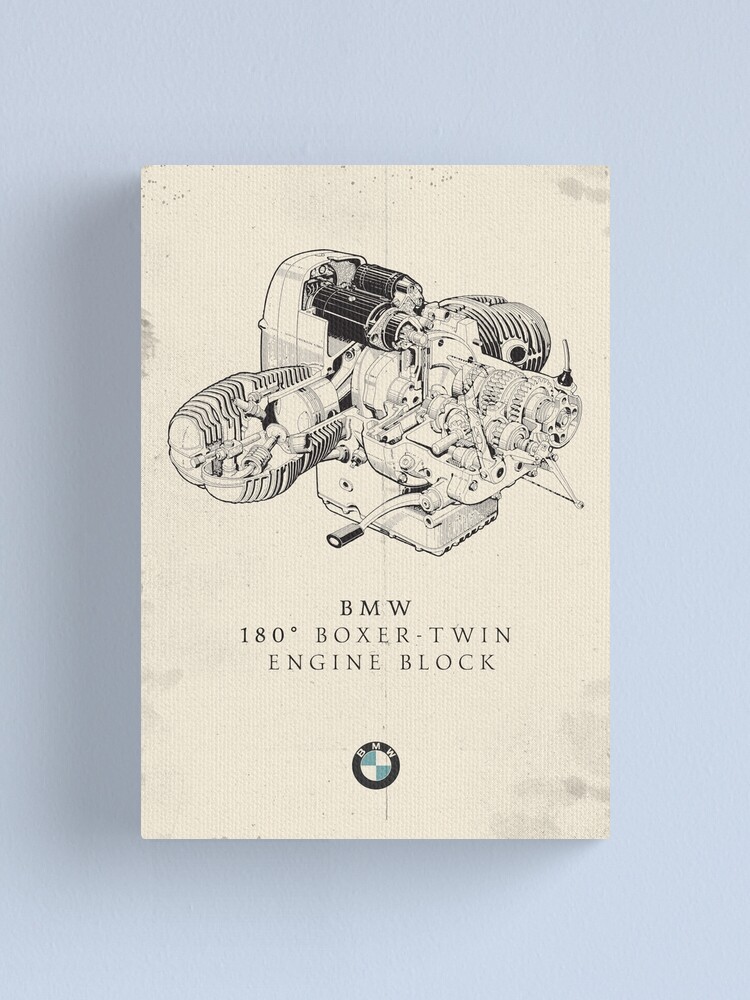The image features an antique automotive service manual by BMW, positioned against a grayish blue background. The off-white, age-worn cover displays noticeable grease smudges and oily fingerprint marks, particularly in the bottom right corner. Centered on the cover, printed in black text, are the words "BMW 180 degrees Boxer Twin Engine Block." Above the text is a detailed black and white illustration of the BMW Boxer twin engine, showcasing its inner workings in a cutaway view. At the bottom of the manual, the iconic BMW logo is prominently displayed in blue, white, and black. This meticulous photograph captures the essence of an old and well-used manual for a BMW 180 degrees Boxer twin engine block.